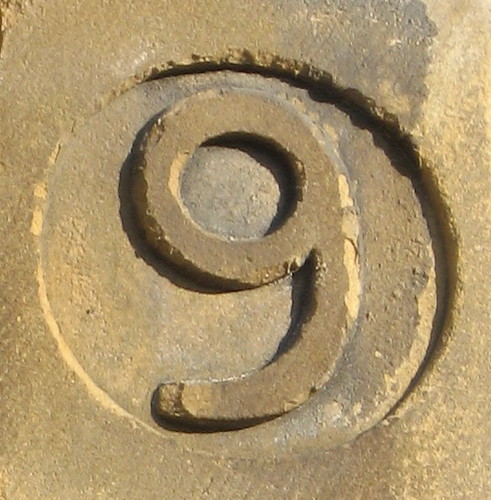The image depicts an aged, dark gray concrete slab, evidently weathered with numerous chips and indents. At the center of the slab, a bold and prominently raised number 9 is encircled by an indented ring, indicating it was stamped into the concrete while still wet. The surface appears scuffed and uneven, with lighter gray patches where the concrete has chipped away over time. The entire piece has a brownish-beige hue with darker stains on the right side, suggesting it may be damp or covered in mud. The photograph captures this textured, weather-beaten surface with the camera pointed directly downward, emphasizing the well-defined, though worn, number 9 at its center.